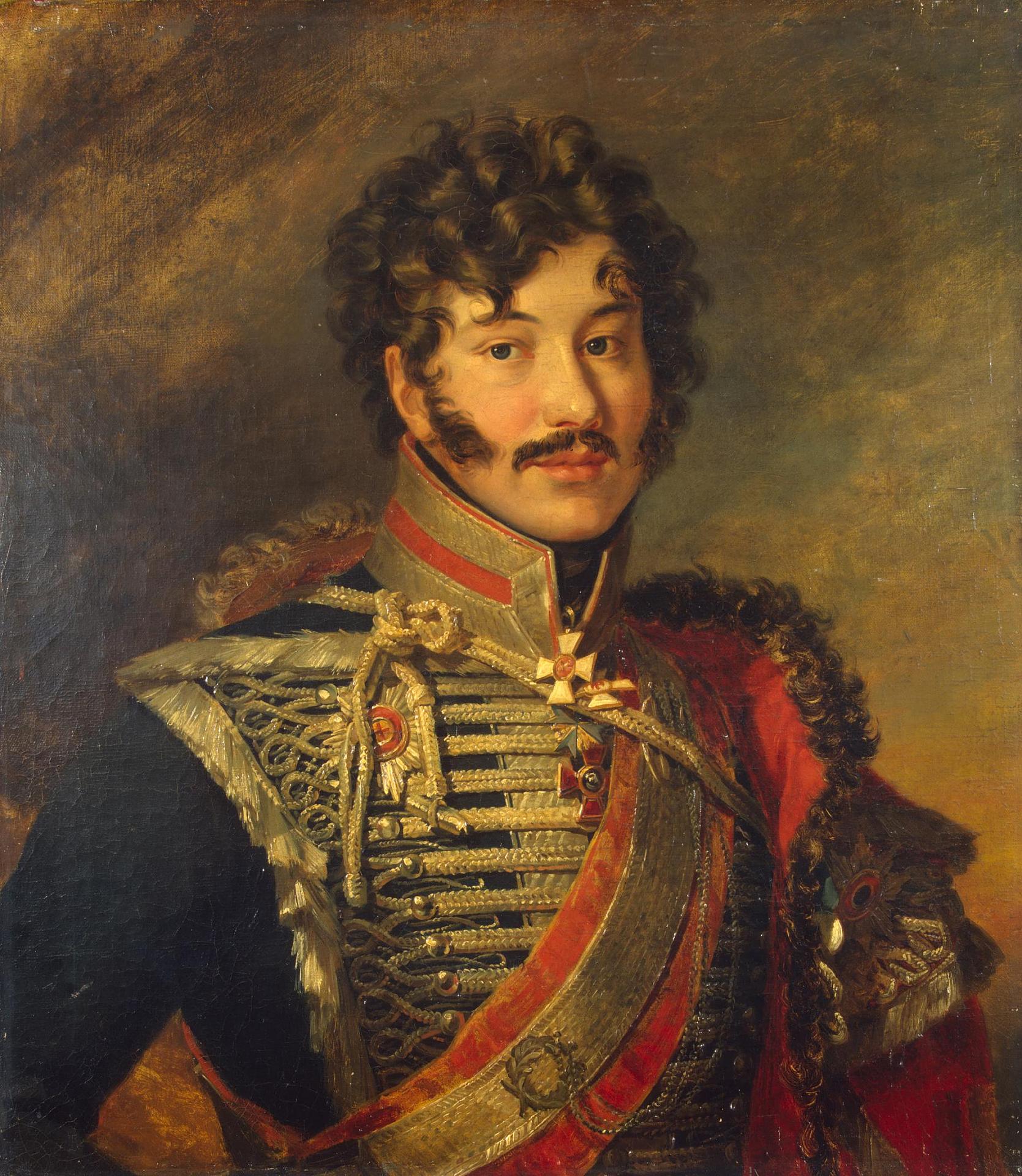The image depicts a historical portrait, likely a hand-painted work, of a young military figure dressed in an ornate, possibly British, uniform. The man has curly brown hair, prominent sideburns, a mustache, and blue eyes set within a face framed by rosy cheeks. His attire is elaborately detailed with tones of navy blue, gold, and red, featuring distinctive elements like a red sash and multiple crosses adorning his collar and chest. The uniform includes a prominent fur trim on one side and along the collar, complemented by an adorned band of warheads and various medals, some appearing wooden. The background is a shadowy blend of brown and green, providing a muted, but rich contrast to the figure’s striking outfit.